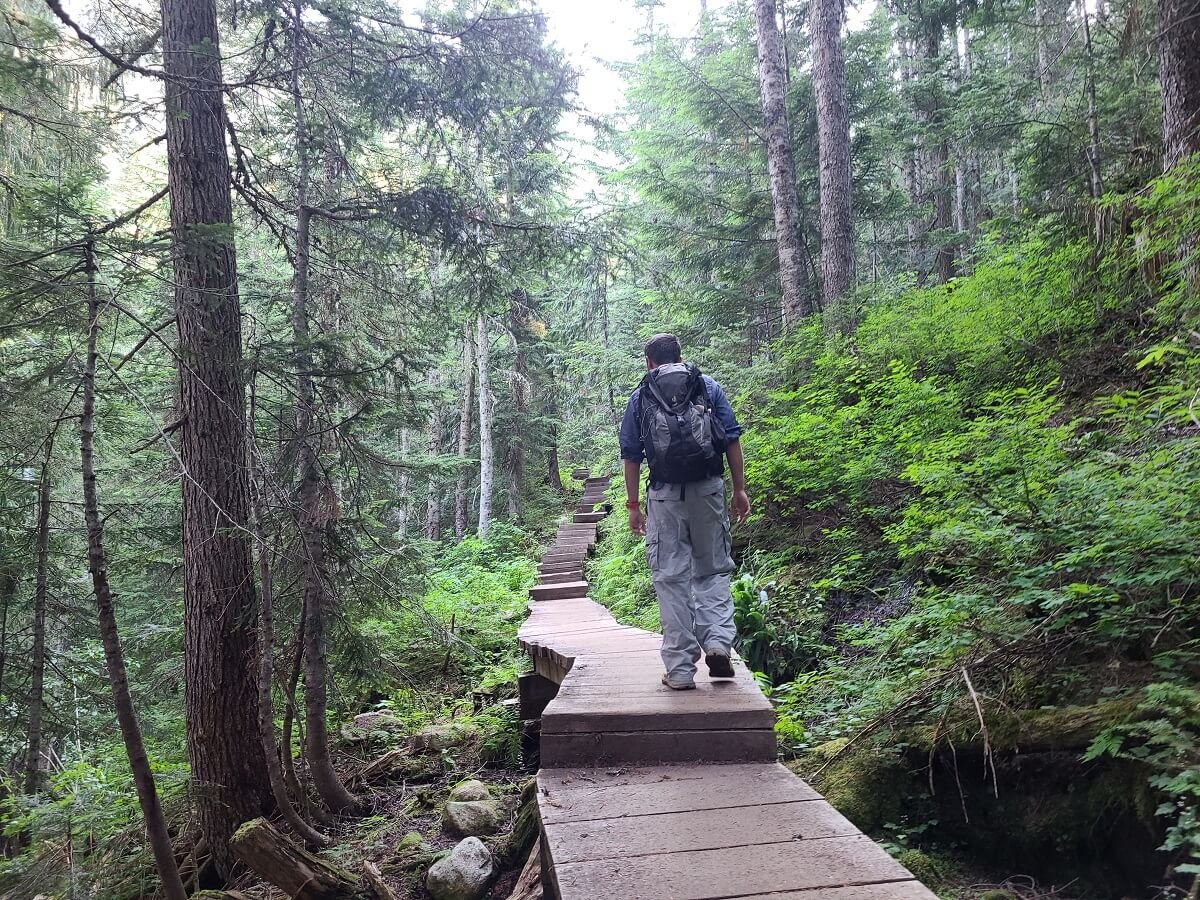A man is captured walking along a narrow wooden pathway winding through a dense forest. The pathway, composed of wooden planks, features steps and elevation changes, leading up a hill to his right and sloping downward to his left. He is dressed in light gray pants, black tennis shoes, and a blue shirt with sleeves rolled up above his elbows, with a grey backpack and a baseball cap on his head. From behind, we see his arms hanging naturally by his sides. The forest surrounding him is lush with tall, branchless pine trees and green undergrowth, indicating a spring or summer setting. Bright daylight filters through the canopy, casting a serene, dappled light on the scene. The wooden path in front of him curves gently to the left and then right, eventually ascending a flight of steps that disappear into the distance.